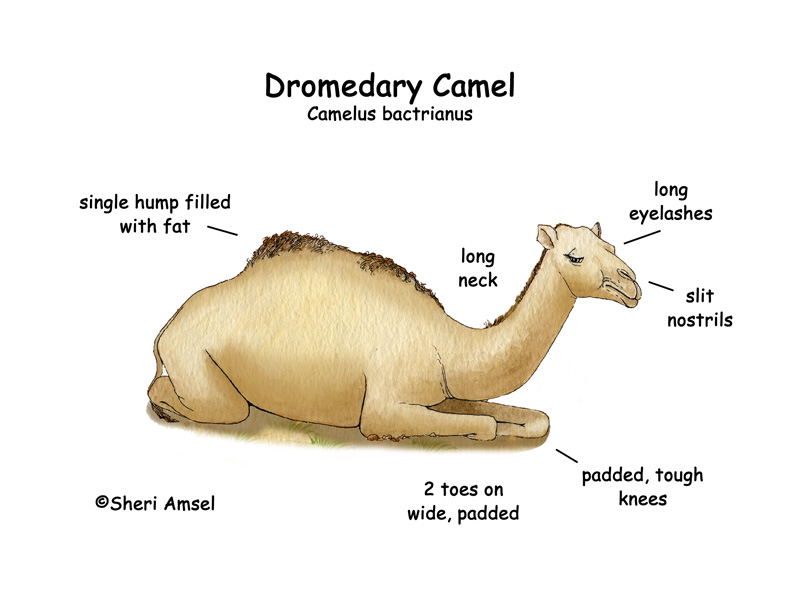In this square portrait image with a completely white background, a central drawing of a light brown dromedary camel captures the viewer's attention. The camel, slightly turned to the left, is laying down on its belly with its head raised and one eye looking downward. At the top middle of the image, thin black text reads "Dromedary Camel," with "Camelus Bactrianus" written below in slightly smaller letters. Around the camel, various arrows point to different parts of its body with descriptive labels. An arrow pointing to its hump reads "Single hump filled with fat," while another pointing at its neck states "Long neck." The caption "Long eyelashes" is directed towards its eye, and "Slit nostrils" points to its nose. Additionally, a label near its legs says "Padded tough knees," and another mentions "Two toes on wide padded feet." The camel is depicted in a cartoonish style, emphasizing an educational purpose for the artwork. Brown, white, black, light brown, and green are the dominant colors in this detailed and intricately labeled illustration. Below the camel's back legs, the artist Sherry Amsel's name and the copyright symbol are visible.